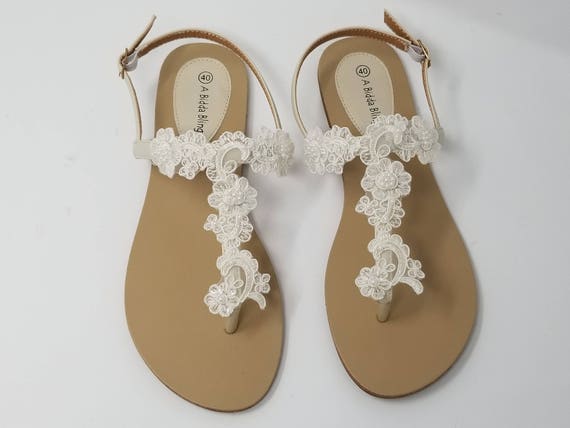This is a detailed color photograph of a single pair of women’s gladiator-style sandals, positioned side-by-side against a plain white background. The sandals feature a flat, tan sole with a distinct oval-shaped patch at the heel that bears the size “40” and the brand name "Abada Bling" in black text. The sole appears to be made of a light beige or brownish leather. The sandals are designed with a strap that divides the big toe from the rest, similar to a flip-flop, and extends towards the heel. This strap is adorned with white lace flowers and intricate designs, some of which include small beads in the center of the flowers. The sandals also have a light brown leather strap that wraps around the back of the wearer's heel, secured with a buckle on either side. The intricate floral lace design and the detailed craftsmanship suggest both style and comfort.